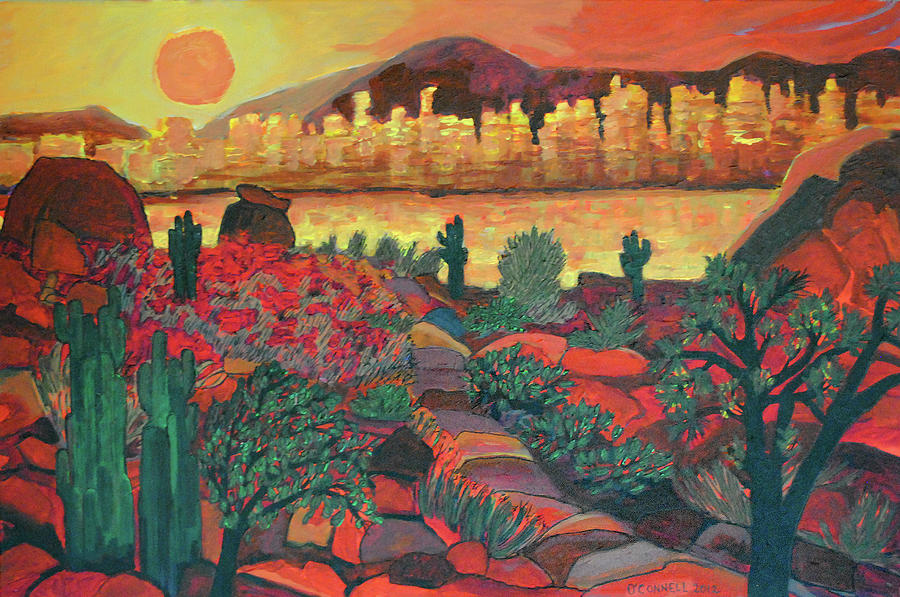The painting features a vividly colored, somewhat impressionistic or cubist depiction of a desert landscape, possibly set in the American Southwest or Mexico. The foreground showcases a variety of flora, including cactus and small trees adorned with red flowers or berries, set among striking red rocks with a tomato-like hue. The terrain here is hard to discern, as it alternates between elements that suggest either sand or water, shaded in yellow and orange tones. Rising prominently in the background are jagged, spire-like orange rock formations, reminiscent of those in Bryce Canyon. Dominating the horizon is an orange sun, either setting or rising, casting a warm glow across the sky filled with yellow and orange hues. There is also a vague, human-like figure assembled from the rocks in the foreground, though it's unclear whether this is an actual person or simply a natural formation. The overall scene captures a dynamic vista of a desert area, rich with diverse shapes and vibrant, contrasting colors.